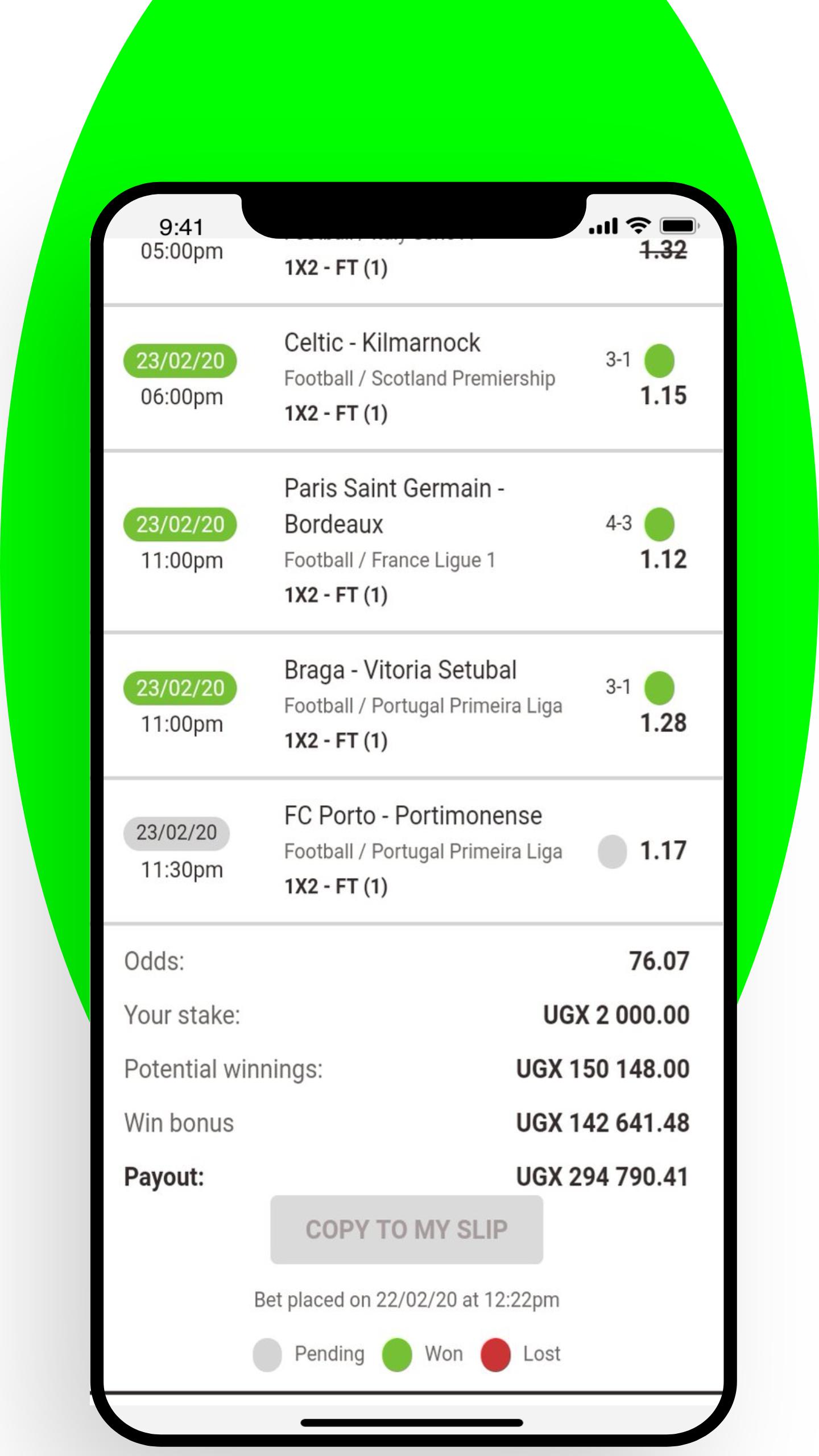In this detailed image, a smartphone is displaying an online betting or gambling app, specifically focused on soccer games. The app's page, which has a white background and black text, lists four different soccer teams: Celtic, Paris Saint-Germain, Varaga, and FC Portal. Each team is categorized by their respective leagues, such as the Scottish Premiership for Celtic, the French Ligue for Paris Saint-Germain, and the Portuguese League for FC Portal.

Beneath the teams' names, the app provides critical betting information, including the odds of winning for each team, the stake, potential winnings, a win bonus, and the total payout. The phone, clearly outlined in the image, rests on a bright lime green oval shape, making the screen's content the focal point of the picture.